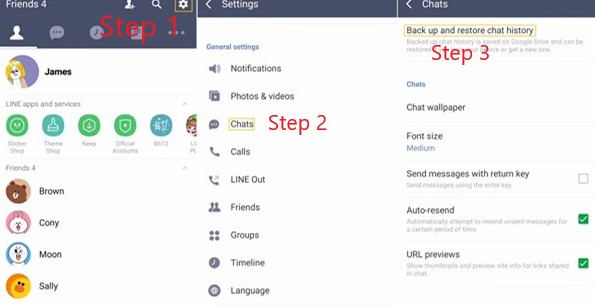The image features a three-step guide on how to backup and restore chat history within a messaging application. 

The first screenshot, marked as "Step 1" in red, showcases a friends list where the user's name is James, along with four contacts: Brown, Coney, Moon, and Sally. For demonstrative purposes, there is a yellow box highlighting the settings gear icon situated at the top right corner.

The second screenshot, labeled "Step 2" in red, highlights the chat option within the settings menu. This menu includes various options such as Notifications, Photos and Videos, Chats, Calls, Line Out, Friends, Groups, Timeline, and Language, with the chat option encased in a yellow box.

The final screenshot, marked "Step 3" in red, directs attention to the "Backup and Restore Chat History" option at the top, which is also highlighted in yellow. Below this option, the menu features additional settings such as Chat Wallpaper, Font Size, Send Messages with Return Key, Auto Resend, and URL Previews.

Together, these images serve as a step-by-step tutorial for users aiming to backup and restore their chat history by navigating through the settings menu—starting from clicking the settings icon, selecting the chats option, and finally choosing the "Backup and Restore Chat History" function.